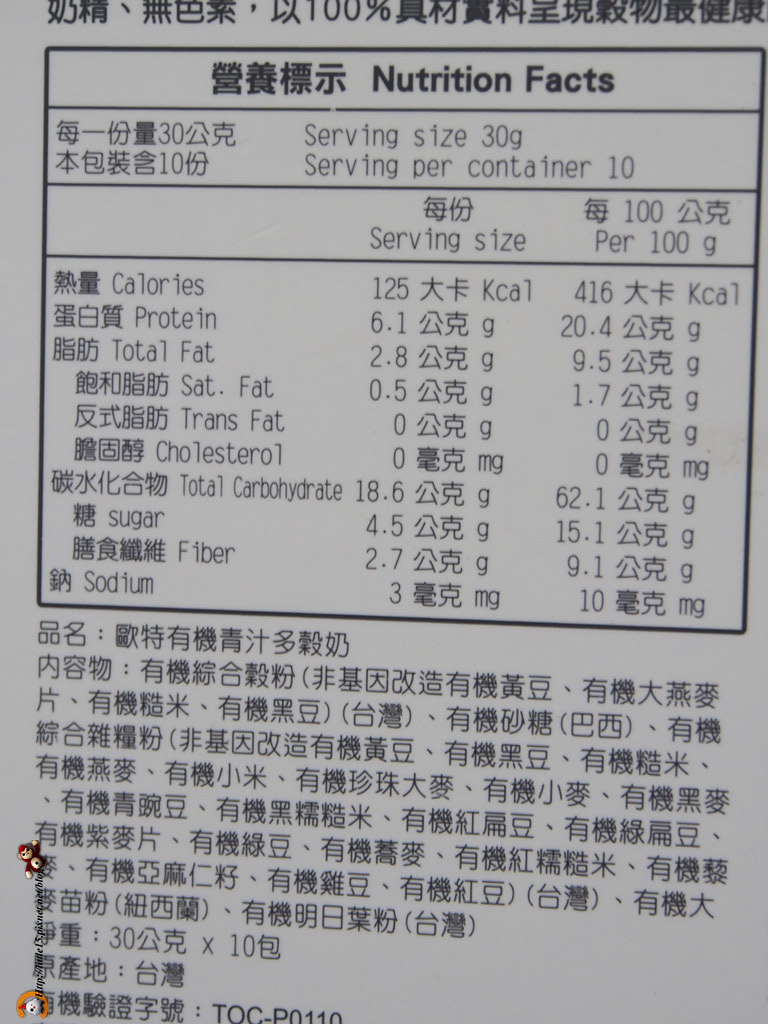This image captures the nutritional facts label of a product, predominantly written in what appears to be Korean, although the exact language is not specified. At the top center of the label, there is a string of Asian characters followed by a rectangular box that contains the heading "Nutrition Facts" in English along with several Asian characters to its left.

Beneath the main heading, the nutritional details are listed, including serving size and servings per container. Specifically, it notes a serving size of 30 grams and servings per container 10, along with nutritional information for a 100-gram serving. This section itemizes caloric content, proteins, total fat, saturated fat, trans fat, cholesterol, total carbohydrates, sugar, fiber, and sodium, each appearing in two columns of numerical values. Corresponding Asian characters are placed to the left of each English term.

Under this detailed nutritional breakdown, a large paragraph is displayed, likely containing the product's ingredient list, which is entirely written in a foreign language assumed to be Asian in origin.

In the bottom left corner of the image, two small icons are overlaid: one depicts a tiny monkey or gorilla, seemingly hanging in motion, and the other is an orange circle with a white shape inside that might resemble a cartoon ghost with two eyes and a mouth. There is also a tiny, hard-to-read text fragment that seems to be a URL link, although its exact content is unclear due to its small size and overlapping placement on the image.